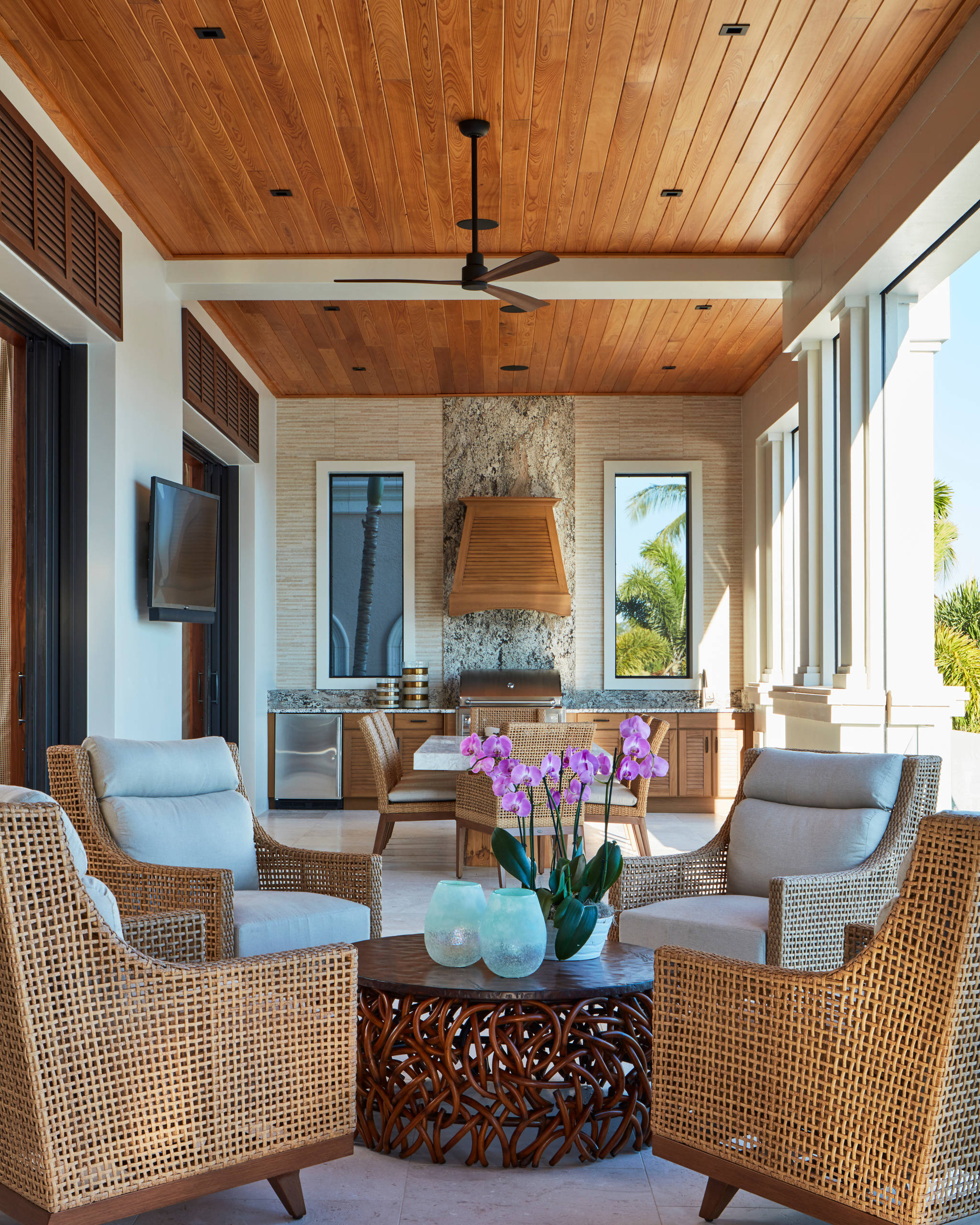This image showcases a beautiful, modern outdoor patio with a wooden ceiling and a large, brass-colored ceiling fan hanging above. The far wall, which features a tan and white tiled design, has two expansive windows. One window, adorned with palm trees, bathes the room in bright light, while the other offers a partial view of another house. A third of this wall is covered in stone, with an exhaust hood clad in wood centered above a stainless steel grill below. 

The counter, running the length of the back wall, hosts a dishwasher and cabinets. To the left wall hangs a flat-screen TV, complementing the modern aesthetic. In the patio center, there are two distinct areas for seating: one with a white marble dining table surrounded by six rattan and cloth chairs, and another conversational space featuring a round, brown table with a cane base and four rattan chairs with white cushions.

Adorning the round table are vibrant purple flowers in a white planter, accompanied by two frosted glass candle holders. The sleek white tile flooring extends towards the right side, which opens to the outside through screened-in columns providing an airy feel. Additionally, two doorways in the right wall lead back into the house, seamlessly blending indoor and outdoor living spaces.